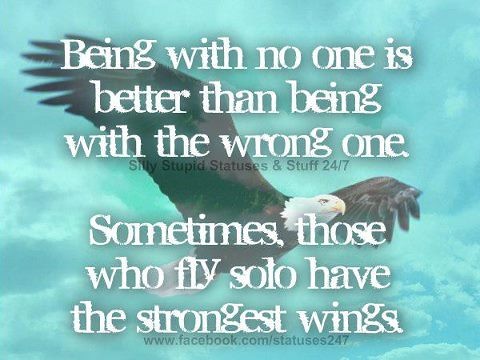This image features a striking depiction of a bald eagle with a majestic white head and yellow beak, soaring through a turquoise blue sky with faint white clouds. The background, though slightly out of focus to emphasize the text, adds a sense of freedom and grandeur. Across the image, a thought-provoking quote is overlaid in a typewriter-style white font with letters unevenly aligned, adding a touch of rustic charm. The text reads: "Being with no one is better than being with the wrong one." Below this, in a separate line, it states: "Sometimes those who fly solo have the strongest wings." In gray font, the image credits "Silly Stupid Statuses and Stuff 24-7" and a Facebook page "www.facebook.com/statuses24-7." The entire composition effectively merges the powerful symbolism of the soaring eagle with motivational text, creating an inspiring visual message.